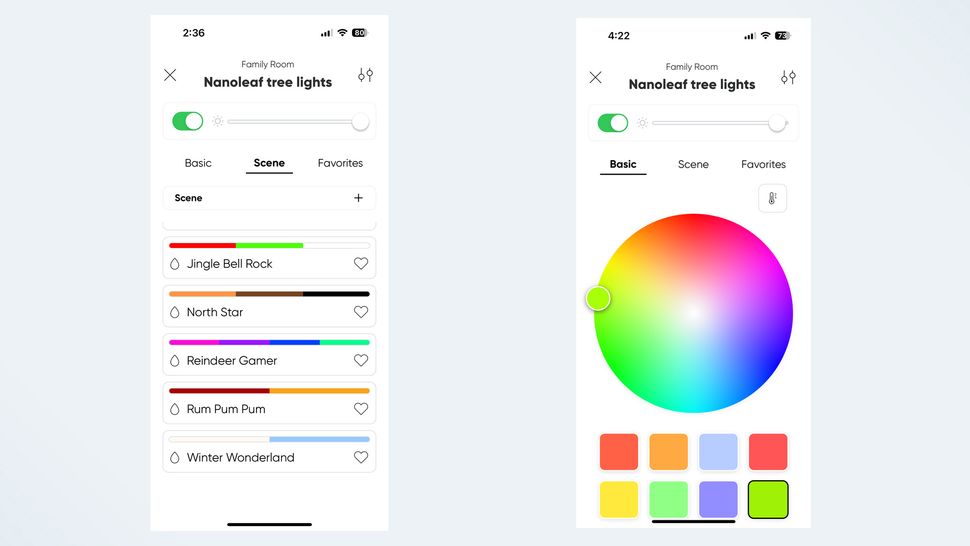The image displays two screens of a smartphone interface in portrait mode. 

### Left Screen:
- **Top Section:**
  - Time displayed in the top left corner as "2:36".
  - Top right corner shows the Wi-Fi, signal reception, and battery icons, with the battery at 80%.
- **Main Display:**
  - The heading "Family Room" is in gray text.
  - Below, in black text, it states "Nanoleaf Tree Lights".
  - An "X" icon is on the left side, and there are small lever icons on the right.
  - Beneath that, there's a green slider button that appears to be on, with a small sun icon next to it. A white marker is positioned all the way to the right, indicating maximum brightness.
- **Scene Selection:**
  - Tabs labeled "Basic", "Scene", and "Favorites", with "Scene" underlined.
  - Scene options listed from top to bottom:
    - "Jingle Bell Rock" with red and green colors.
    - "North Star" with yellow, orange, brown, and black colors.
    - "Reindeer Gamer" with pink, purple, blue, and green colors.
    - "Rum Pum Pum" with brown and yellow/orange colors.
    - "Winter Wonderland" with white and blue colors.

### Right Screen:
- **Main Display:**
  - A large central circle filled with various colors.
  - A small green circle located on the left side of the large circle.
- **Color Options:**
  - Eight square color swatches are displayed below the circle, each in different colors.